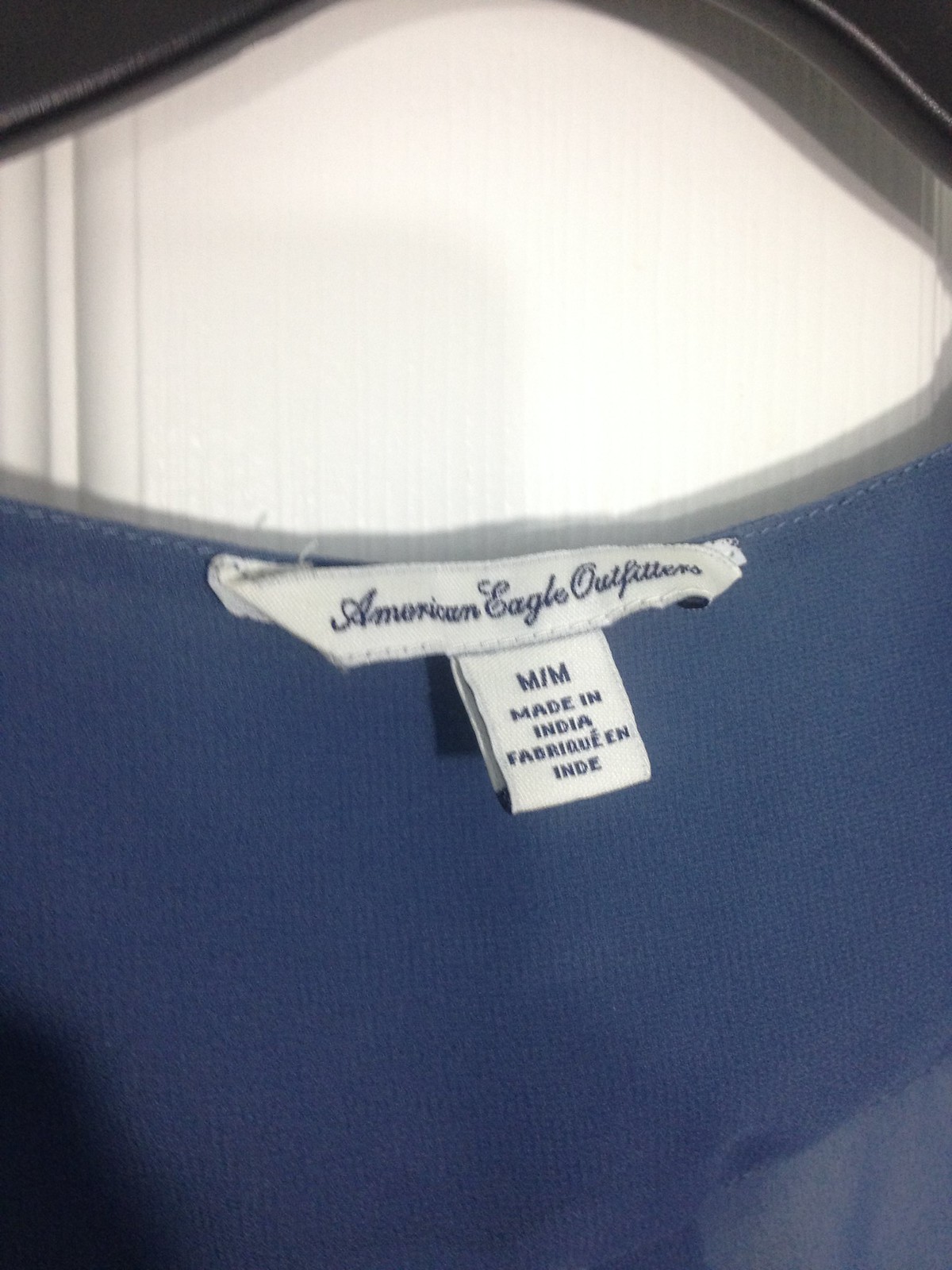Here's a cleaned-up and detailed caption for the image:

"An up-close photograph showcasing the label inside a piece of clothing. The image features black shading in the top left and right corners, framing an oval-shaped area of white outlined in gray. Centered at the bottom of the white oval is a rectangular white tag with 'American Eagle Outfitters' elegantly written in black cursive. Directly below this, a square white tag is visible, featuring 'M/M' in bold black capital letters. Beneath that, the tag notes 'Made in India' along with additional black text. The fabric of the shirt is predominantly blue with shades of gray visible in the lower right corner."